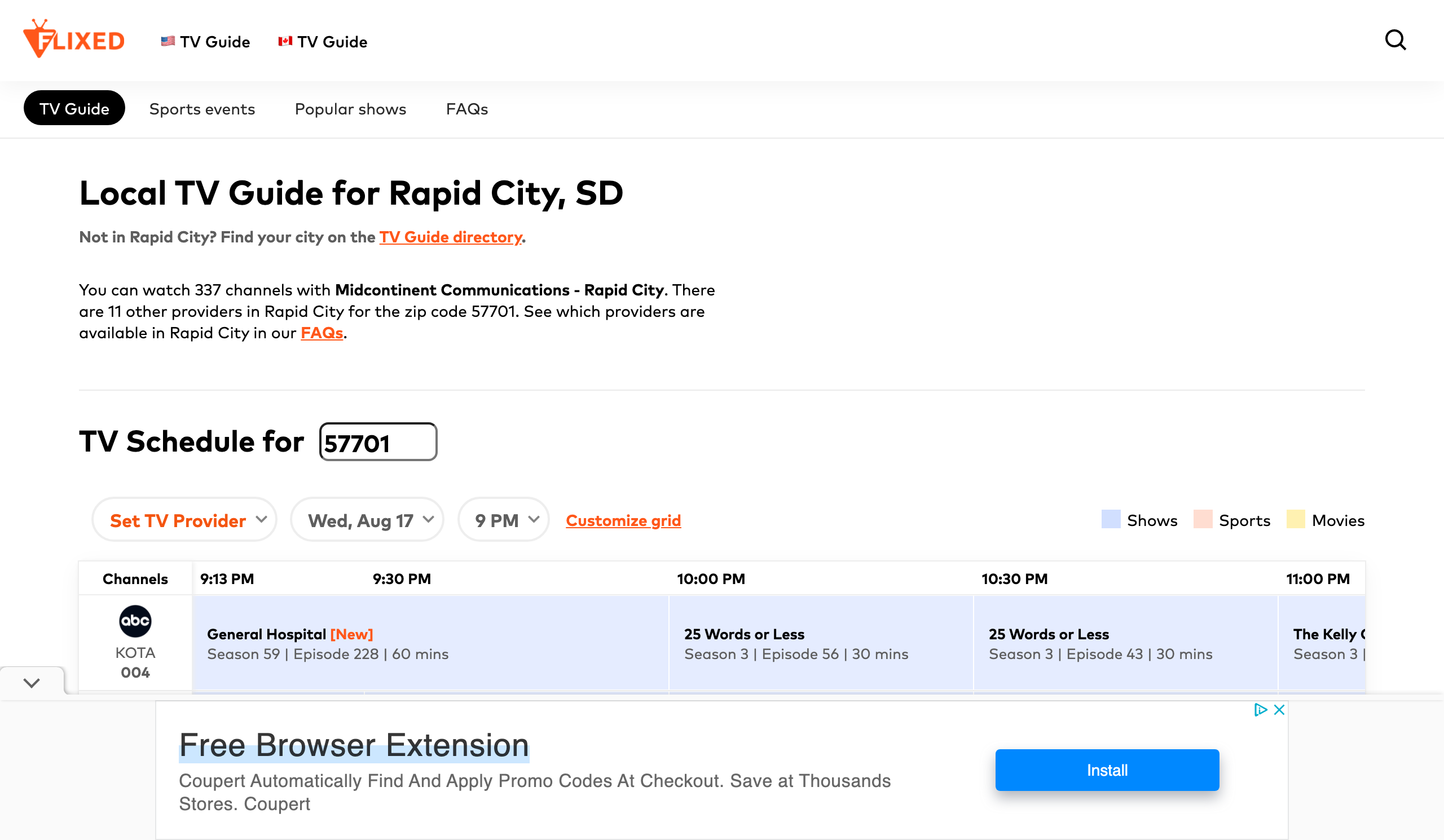This image is a screenshot of the Flixed website, specifically its TV guide section. At the top, there's a white menu bar where the word "Flixed" is displayed in orange text on the left-hand side. Next to it, there are two TV guide options: one with an American flag and the other with a Canadian flag. To the right, there's a search bar. Below the main menu, there are several navigation options displayed horizontally. The "TV Guide" option is highlighted in a black oval, while the other options—"Sports Events," "Popular Shows," and "FAQs"—are listed normally.

Underneath the menu, black text reads "Local TV Guide for Rapid City, SD," followed by "Find your city on the TV guide directory," with the words "TV guide directory" formatted as a clickable orange hyperlink. Below this, text explains that you can access information for 337 channels with Midcontinent Communications in Rapid City, noting there are 11 other providers available for Rapid City's zip code, 57701. The phrase "see which providers are available at Rapid City in our FAQs" includes "FAQs" as another clickable hyperlink.

Further down, the text "TV Schedule for" is displayed next to a box containing the zip code "57701." The interface provides options regarding the TV provider and the date, which is specified as Wednesday, August 17, 9 p.m. There are also options to customize the viewing grid.

A search result is displayed below, beginning with the channel listing for ABC, labeled as KOTA, channel 004. At 9:13 p.m., the program "General Hospital" is scheduled, noted as a new episode from season 59, episode 228, with a duration of 60 minutes. This is followed by the listing for the next program, "25 Words or Less."